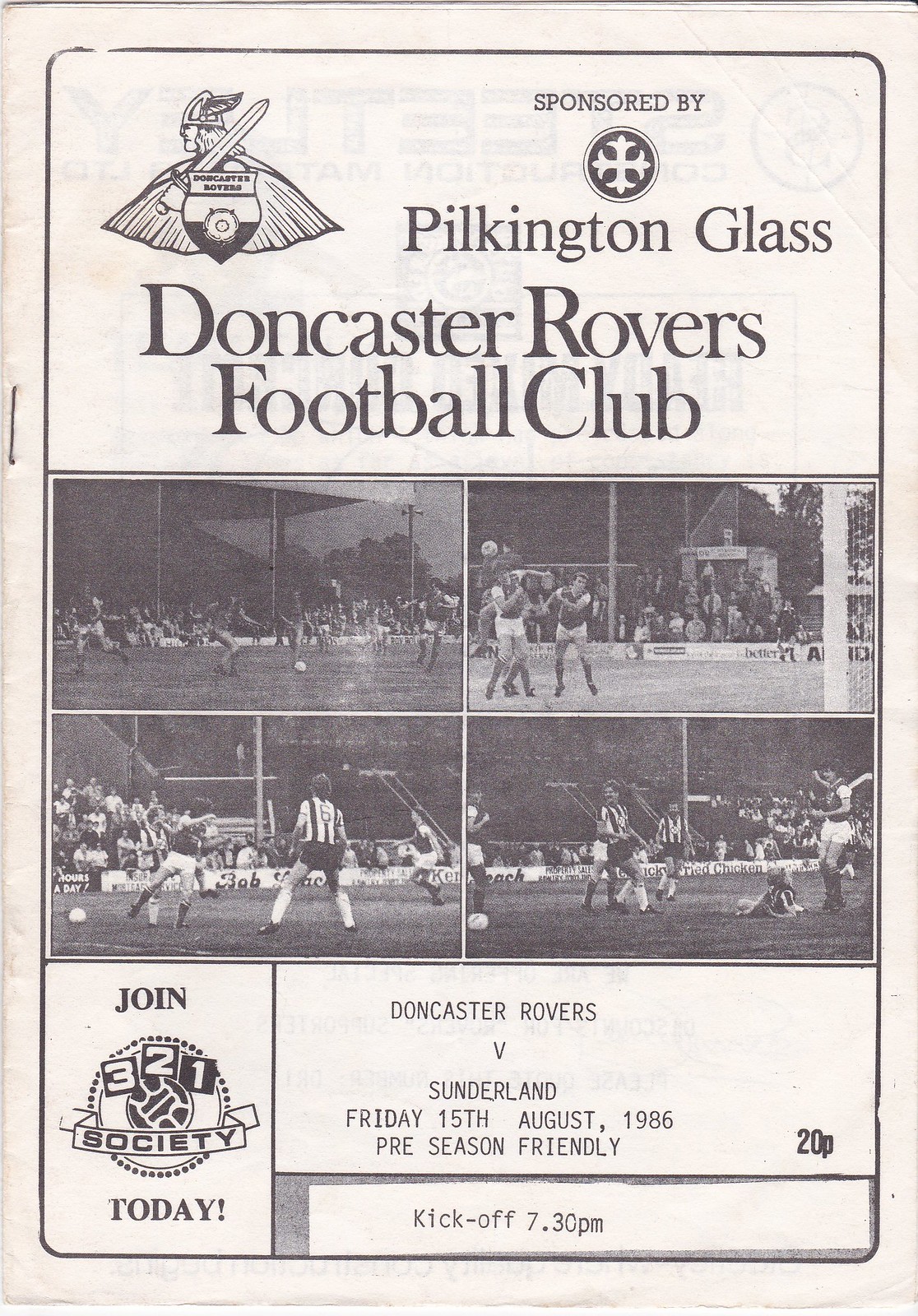This tall, rectangular image depicts the front page of a sports program for a preseason friendly match. The off-white paper is somewhat bent and wrinkled at the edges, with a staple just above the center on the left side. Enclosed within a black thin border – rounded at the corners – the upper left corner features a black and white Viking symbol, showcasing a Viking facing left, wearing a helmet with wings, a cape, and holding a sword and shield. To the right of this emblem, it reads "Sponsored by Pilkington Glass" and "Doncaster Rovers Football Club." Centered below, four wide black and white photographs depict soccer players in action, arranged in two rows. Further down, various advertisements and text reside, including the call to action "Join 3-2-1 society today" in the bottom left corner. The bottom right corner details the event: "Doncaster Rovers v Sunderland, Friday 15th August 1986, preseason friendly, 20p," followed by "Kickoff 7:30 p.m." This flyer provides comprehensive information about the upcoming match while showcasing relevant soccer imagery.